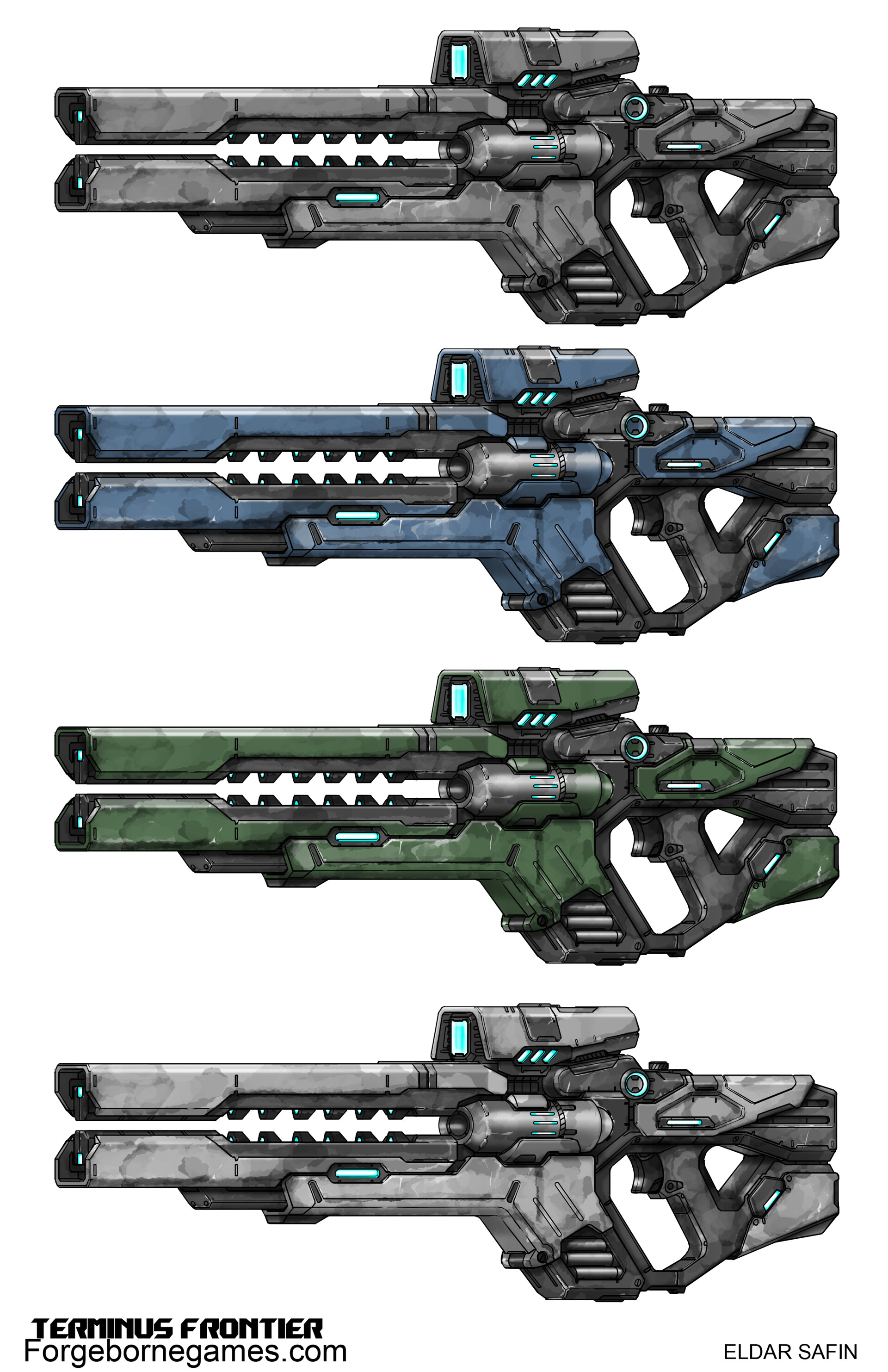This image is an advertisement showcasing four futuristic gun skins from the game "Terminus Frontier," available at ForgeBorneGames.com. The skins are copyrighted by Eldar Safin. The guns are arranged vertically, with each skin in a distinct color: gray, blue, green, and silver. Each gun is equipped with two front prongs and a scope on top, giving them a high-tech, possibly paintball-like appearance. The design includes canisters on the side and features reminiscent of a dinosaur mouth, enhancing their unique, futuristic appeal.